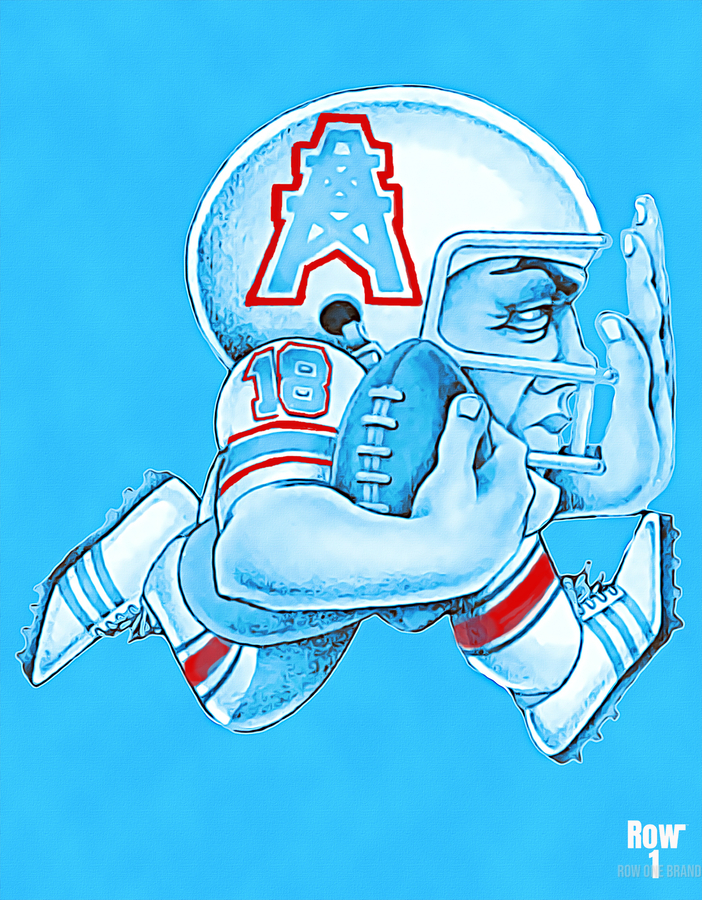This image is a highly stylized and artistically altered illustration of an American football player in action, rendered in a cartoon-like manner with a predominantly blue color scheme. The player, a striking figure with an exaggeratedly large head, is captured mid-dive clutching a football securely against his side. The athlete's helmet, adorned with a team logo that resembles a red letter 'A' with a star, enhances its patriotic American flair. The player wears a football uniform with the number 18 prominently visible on the jersey, which features red and white stripes on the sleeves. His body is depicted in a dynamic pose, running to the right, with his right leg extended forward and left leg back, giving an impression of swift motion. Intricate details like the stripes on his socks and shoes, and the expressive features of his face—eyebrows, eyes, nose, and lips—show through his helmet, adding to the surreal and detailed aesthetic. In the bottom right corner of the baby blue background, white text reads "Row 1," with a faint "Row 1 Brand" overlaying the number 1, completing this vibrant and detailed illustration.